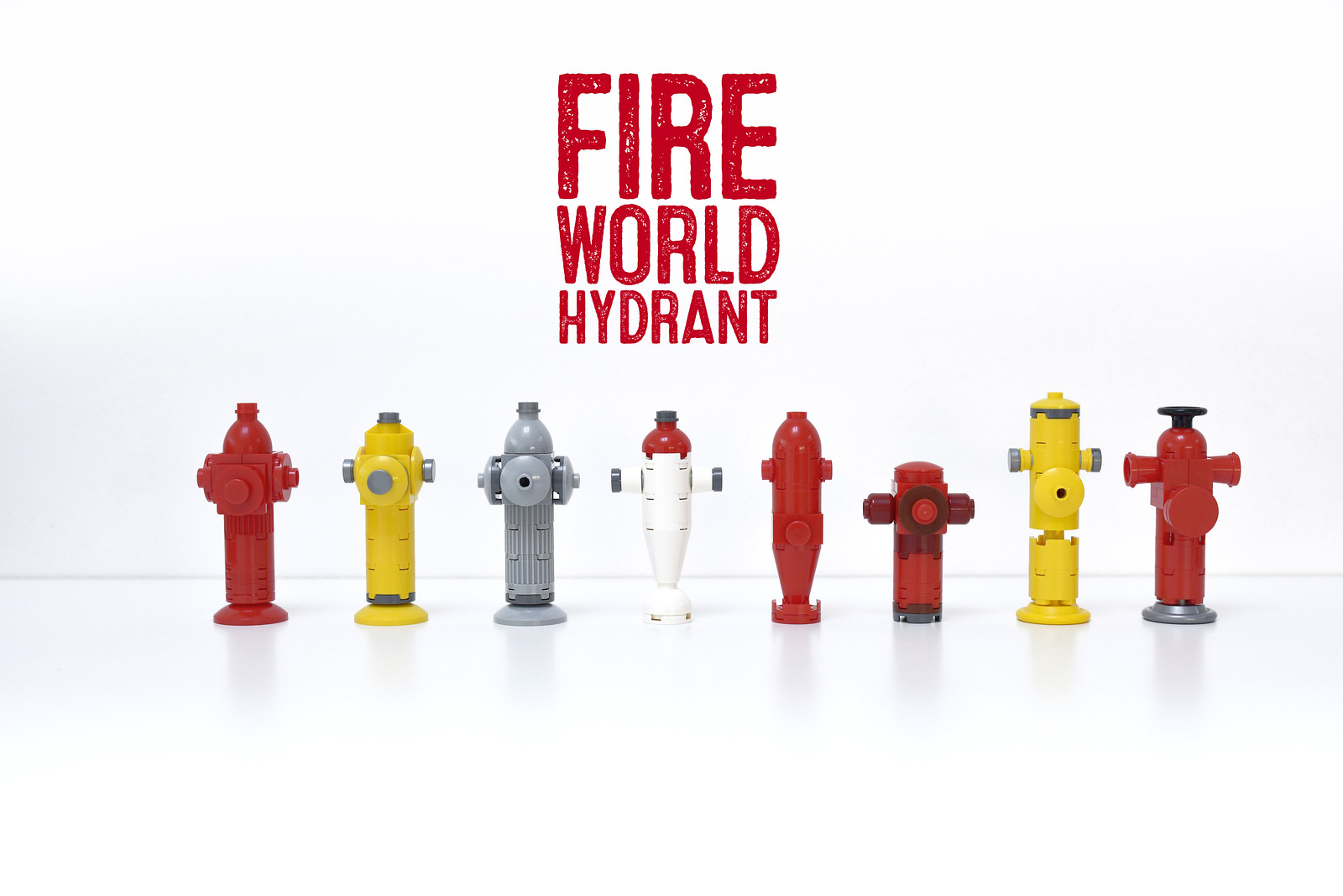This is a photograph showcasing eight distinct fire hydrants, arranged side by side on a slightly reflective white floor with a white background. At the top, red text reads "Fire World Hydrant," featuring white specks within the lettering, giving a promotional feel. On the far left is a classic red fire hydrant, followed by a somewhat shorter yellow and gray hydrant with black accents. Next is a completely gray hydrant, succeeded by a white hydrant with a red top and silver arms. The fifth in line is another fully red hydrant, shiny in appearance. The sixth one is the shortest, a T-shaped red hydrant with extended arms. Next is a taller yellow hydrant with gray tips on its arms and near the top. Concluding the lineup is a red hydrant with a black top and a silver base. Each hydrant varies in shape, size, and color, effectively contrasting against the white background and floor.